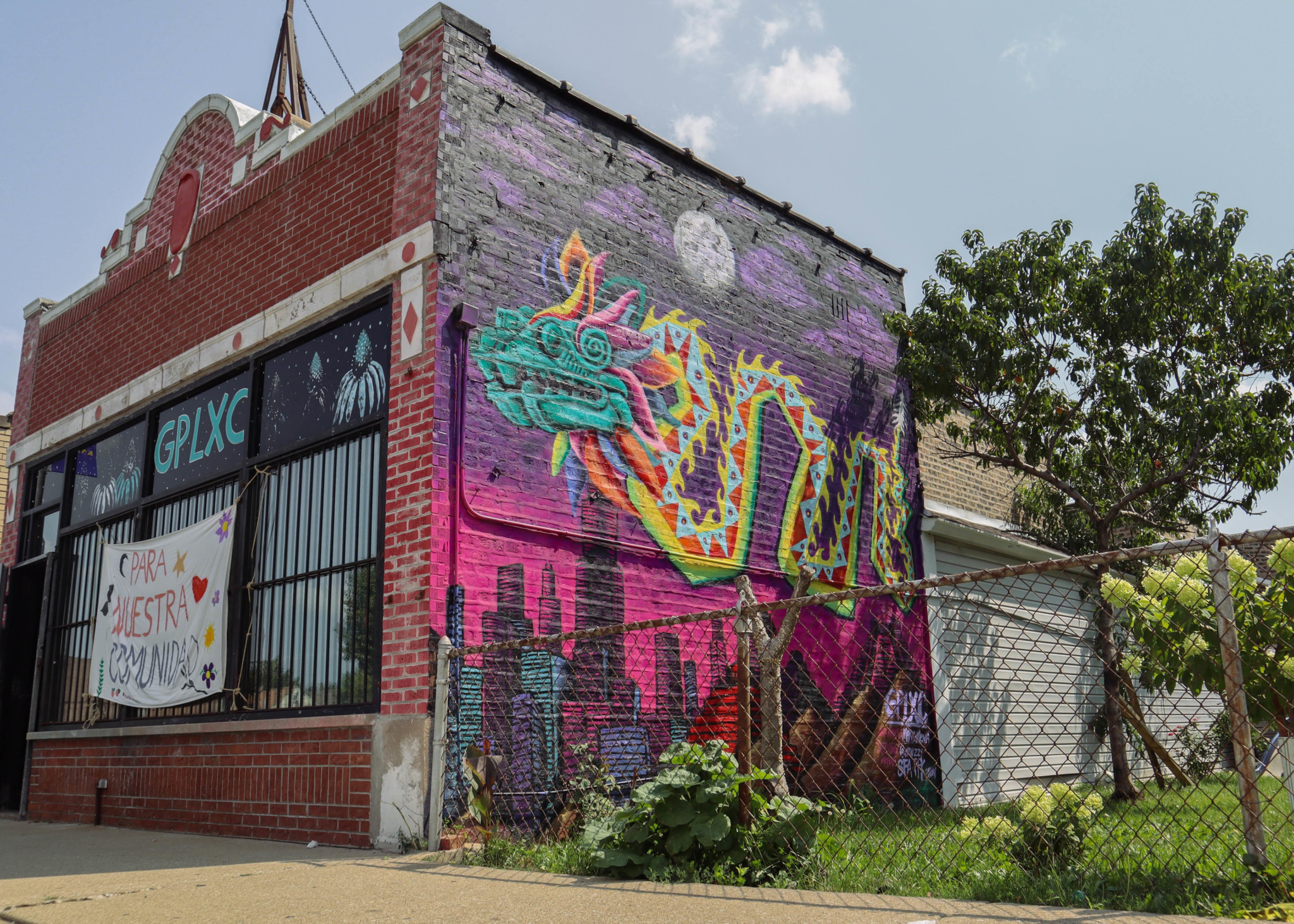This exterior photograph captures an old, one-story red brick building with a commercial façade. The building features black bars on its front windows, some graffiti, and an unknown Spanish sign, hinting it has been there for quite some time, possibly around 100 years. Dominating the side of the building is a large, vibrant mural that serves as the focal point of the image. The mural showcases a magnificent, ornamental eastern dragon with a long serpentine body, adorned in turquoise, yellow, red, and occasionally green. The dragon soars over a painted cityscape under a pink and purple sunset with a prominent moon in the sky. The mural is partially obscured by a chain-link fence situated in front of a fenced-in grassy area with some cactus, which adds to the urban yet slightly overgrown setting. The photograph is taken at an angle that beautifully captures both the front and the side of the building, presenting a comprehensive view of this striking piece of street art.